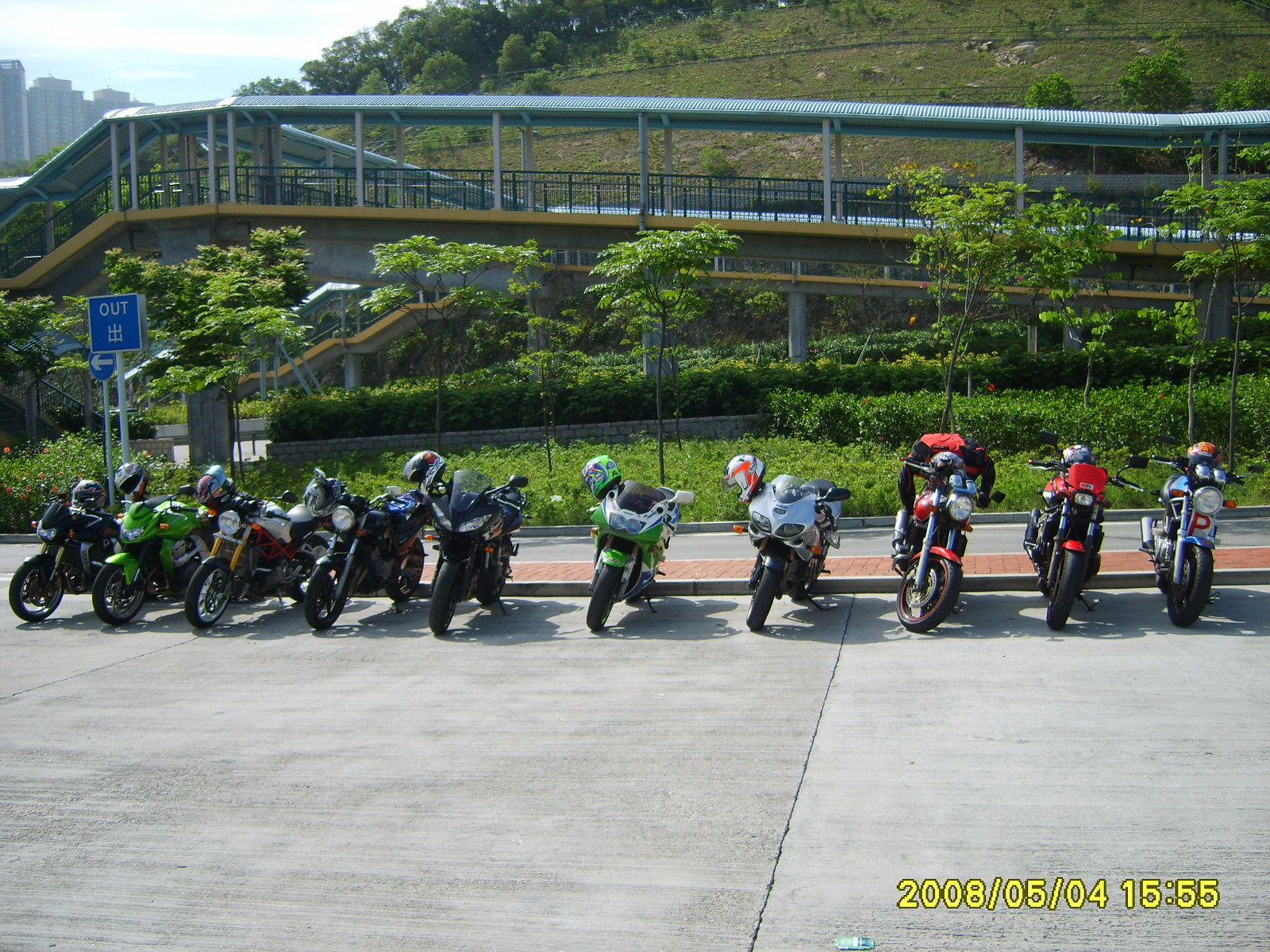This is a color photograph of a parking lot featuring approximately 10 motorcycles lined up next to each other on concrete pavement. The motorcycles vary in size, color, and make, with each one adorned by a helmet resting on its handles. Starting from the right, there's a silver motorcycle marked with a red "P" on the front, followed by a black and red motorcycle, a white and red one, another silver bike with a red helmet, a green and white motorcycle with a matching green helmet, a black motorcycle with a black and white helmet, another black motorcycle with a black helmet, a red, yellow, and black bike with a black helmet, an all-green motorcycle with a yellow and white helmet, and another black motorcycle with a black helmet. There is a timestamp at the lower right in yellow text displaying "2008-05-04 15:55." 

Behind the motorcycles, a paved walkway with green railings and yellow and white borders slopes down from left to right, and it includes a stairway on the far left. Trees line the area between the motorcycles and the walkway, giving way to a green lawn and a sloping hill beyond. Additionally, there is a blue square sign with the word "out" and six dots and a circular blue sign with a white arrow pointing left in the upper left section of the image. In the distant background, there is also a faint hint of a cityscape on the upper left.